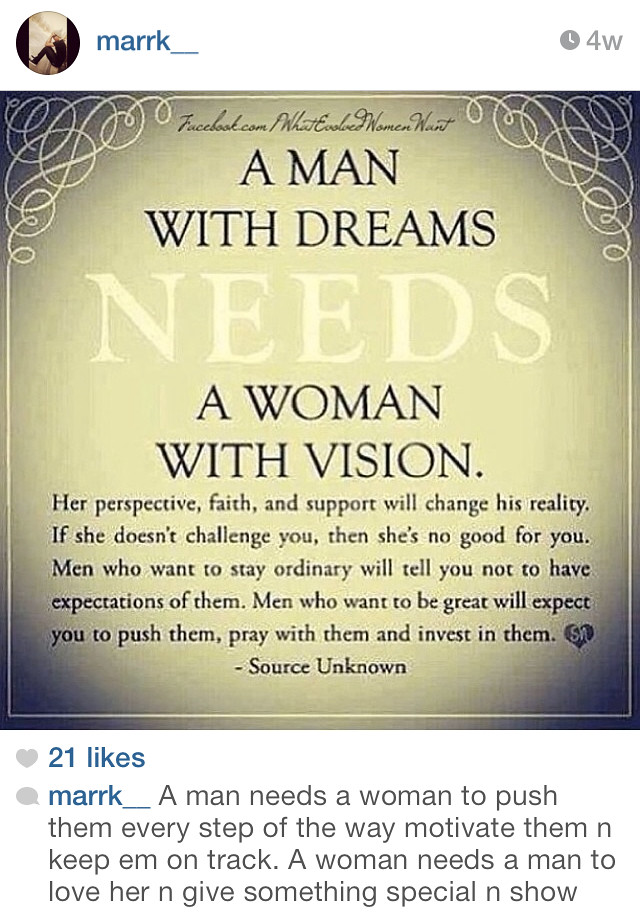This screenshot depicts a social media post, likely from Facebook given the layout, made by the user "Mark_" four weeks ago. The post has garnered 21 likes. At the top left corner, the username "M-A-R-K underscore" is displayed, while the top right corner indicates the time of posting with "4W." The main image features a motivational quote on a golden background with a black border along the edges. The quote reads: "A man with dreams needs a woman with vision. Her perspective, faith, and support will change his reality. If she doesn't challenge him, then she's no good for him. Men who want to stay ordinary will tell you not to have expectations of them. Men who want to be great will expect you to push them, pray with them, invest in them." At the bottom of the image, it's noted to be "source unknown." Below the image is Mark's commentary: "A man needs a woman to push them every step of the way to motivate them and keep them on track. A woman needs a man to love her, give her something special, and show." The quote and commentary reflect on traditional gender roles, emphasizing the supportive and motivating roles expected in relationships.